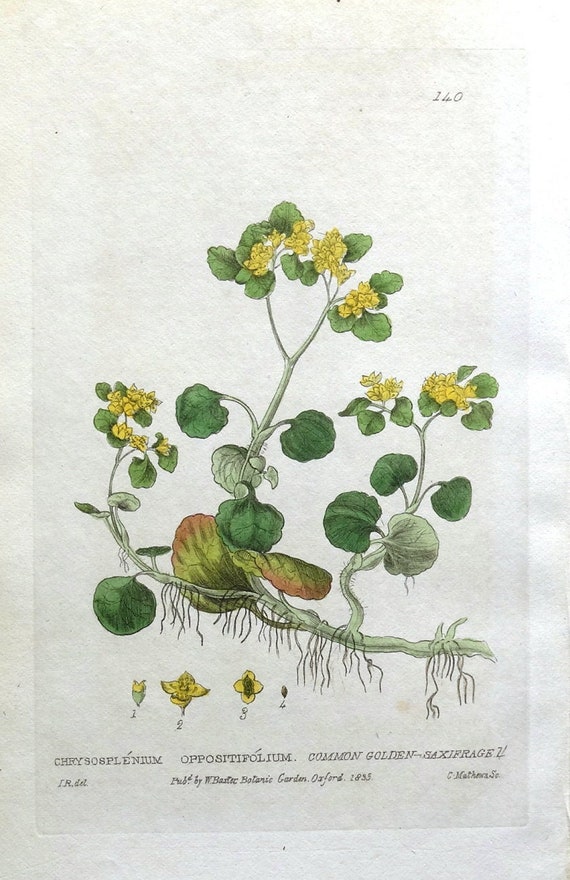This detailed botanical study is a meticulously crafted illustration, likely rendered in pen and ink and enhanced with color. The artwork, which could be on cloth or beige paper, portrays the life cycle of a daisy-like flower named Chrysosplenium, with its Latin labels meticulously inscribed at the bottom. The illustration exemplifies both scientific precision and artistic finesse, depicting the plant from seed to mature flowering stages. Each stage is represented: starting from the seed, progressing to a bulb, then a flowering plant, closing up, and finally becoming a seed again. The plant is characterized by short, light green stems that sprout veiny, dark green, circular leaves. These leaves appear intermittently along the thick, colorful vines. At the top, a tuft of green leaves encircles clusters of small, yellow flowers. The roots, depicted feathery and veiny, reveal the intricate underground structure of the plant. Surrounding these botanical elements, the image includes feathery root-like lines and other branches extending upwards, emphasizing the plant's detailed anatomy.